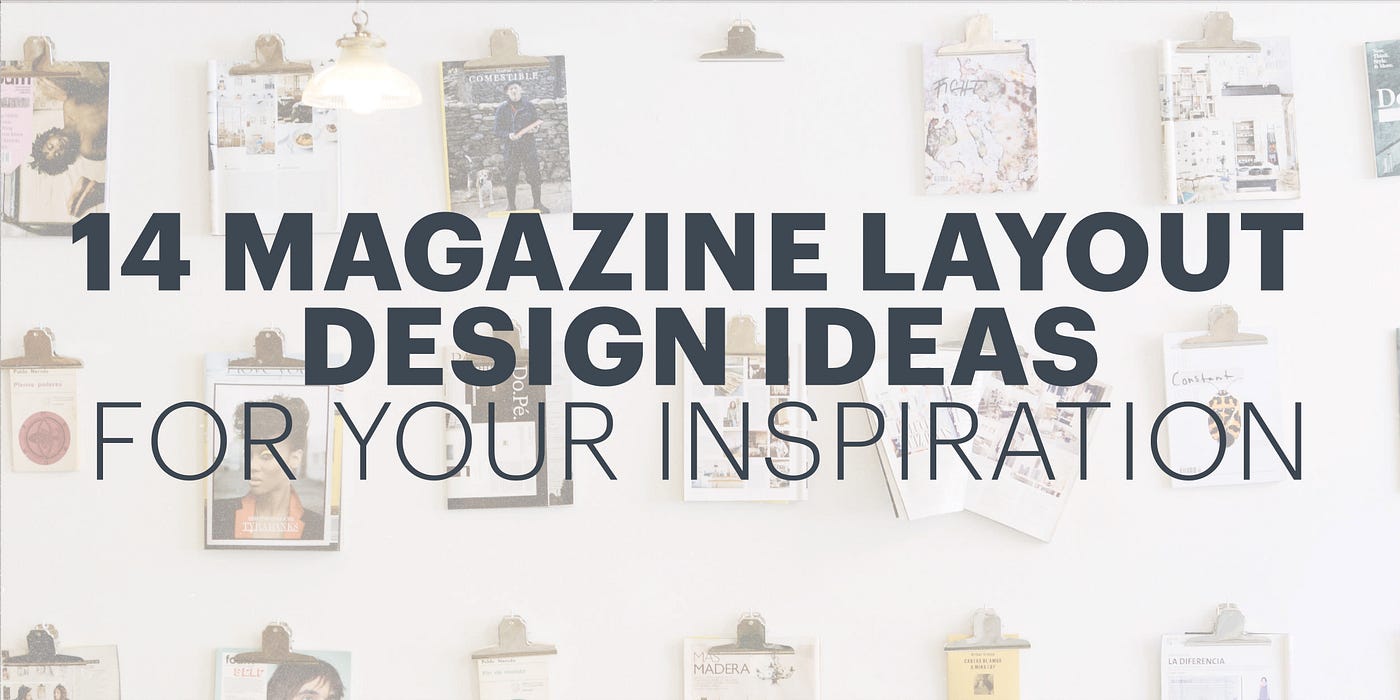The image showcases an array of magazine pages clipped to a white wall in three neat rows, each row featuring five to six pages held by gold clips. The magazines are displayed in a way that either the article or the cover of each magazine is visible, adding a vibrant mix of designs and colors to the composition with noticeable hues of white, yellow, black, and orange. Overlaid upon this backdrop, the image is adorned with bold, capitalized black text that reads "14 MAGAZINE LAYOUT DESIGN IDEAS," followed by a line of thinner black text underneath that states "FOR YOUR INSPIRATION." A hanging lamp from the top of the image illuminates the display, further confirming the magazines are indeed suspended and not laid flat. The overall aesthetic provides a visually inspiring collection of magazine layout examples.